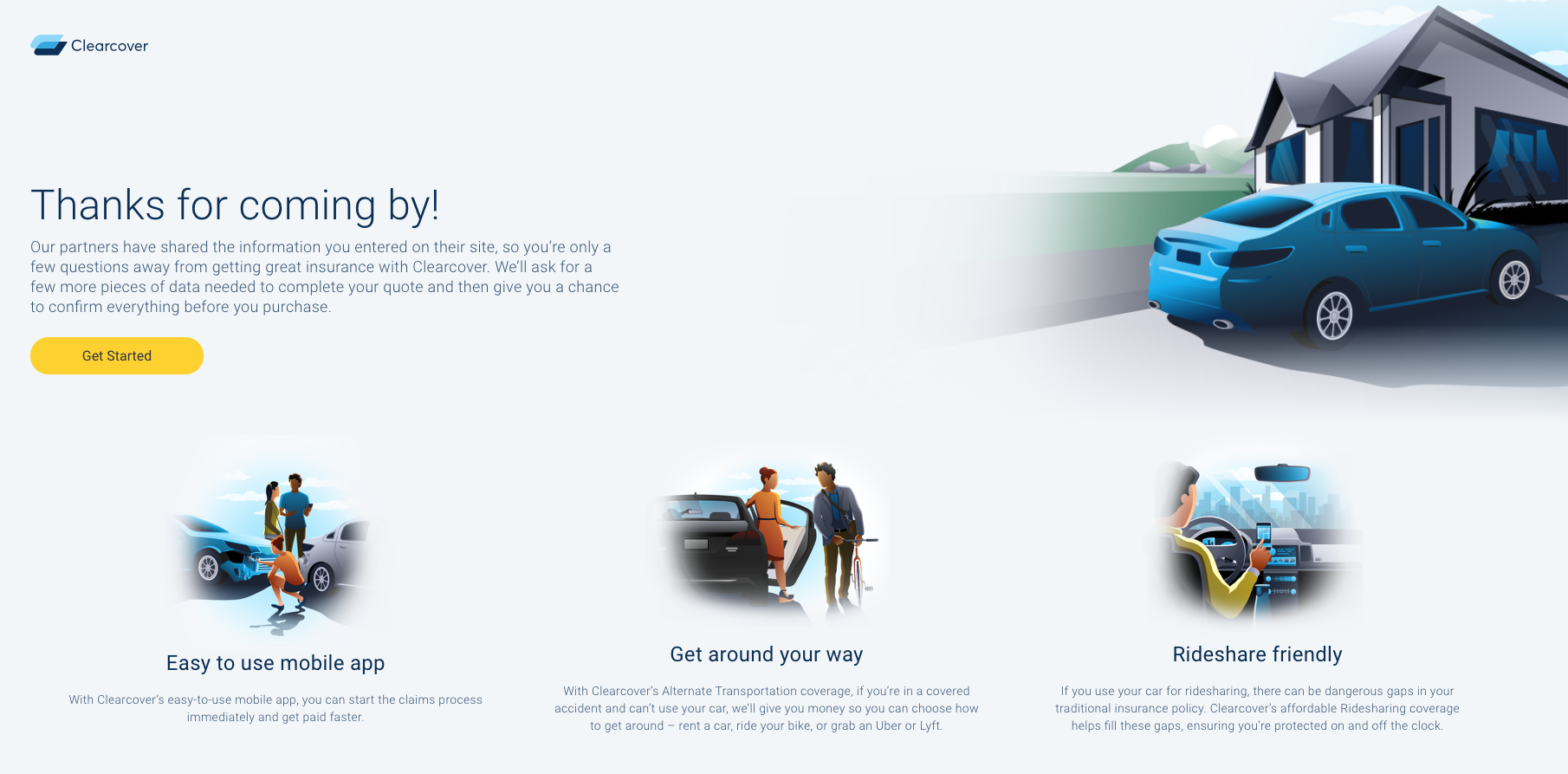This image is a detailed screenshot or promotional graphic with the dimensions of a typical desktop display. It features a light background in the upper left corner, where a design element resembling a glass panel with a dark shadow underneath is visible. Prominently displayed is the product name "ClearCover" written as one word. Below, a welcoming message reads, "Thanks for coming by. Our partners have shared the information you entered on their site. So you're only a few questions away from getting great insurance with ClearCover. We'll ask for a few more pieces of data needed to complete your quote and then give you a chance to confirm everything before you purchase." A conspicuous yellow button invites users to "Get Started."

On the right side, there is a digital illustration showcasing a house with a car parked in front, set against a backdrop of mountains. Three smaller images line the bottom of the screenshot, each depicting people in or around their cars. The first image promotes the mobile app, the second is captioned "Get Around Your Way," and the third indicates the service is "Ride Share Friendly."